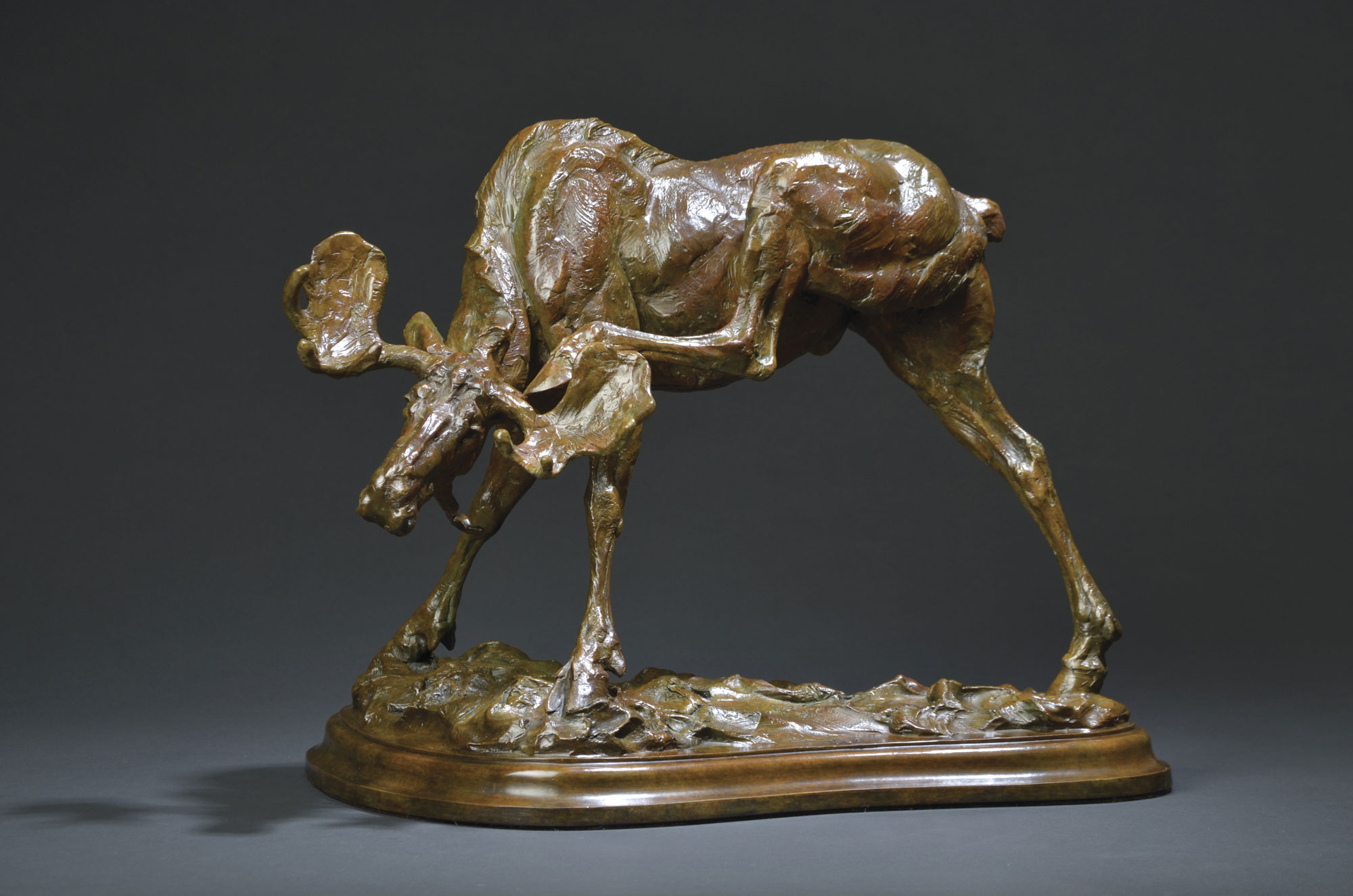This detailed sculpture depicts a moose, possibly crafted from bronze or a bronze-colored material, showcased on a polished wooden base. The moose is captured in a captivating and dynamic pose, standing on three legs while its left hind leg reaches up to scratch behind its large, thick antlers or possibly its ear, creating an intriguing scene. The animal's head is tilted slightly to the left and tucked towards its front thighs, highlighting every sinew, muscle, and tendon in its body with impressive detail, suggesting a moment of concentration and exertion. The sculpture's textured surface indicates the rough terrain the moose is standing on, adding to its realism. Its tail is subtly wrapped to one side, emphasizing the motion and natural posture of the moose. The base of the sculpture is also adorned with a rough bronze or plaster relief, seamlessly integrating the moose into its environment. Overall, this exquisite piece superbly captures a unique moment in the life of a moose, combining realism and artistic expression.